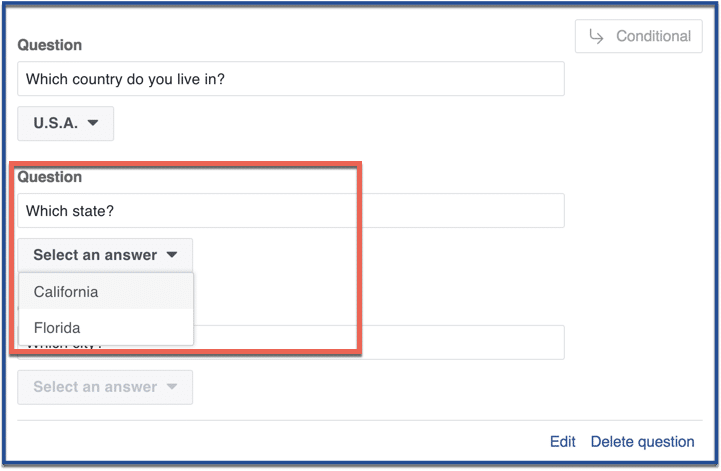The image depicts a screen from a device with a distinct blue border framing a white background. On the top left corner of the screen, there is a rectangle containing an arrow pointing to the right, with the word "Conditional" (spelled out as C-O-N-D-I-T-I-O-N-A-L) following the arrow. On the top right corner, the screen displays the word "Question."

Beneath these elements, a question is posed: "Which country do you live in?" The response "U.S.A." is shown, accompanied by a downward-pointing black arrow. Below this section, there is a red-bordered square. In the top left of this square, it reads "Question," followed by the query "Which state?" under it. Below this query, it says "Select and Answer" with options for "California" and "Florida."

Outside and below the red square, there is a button labeled "Select and Answer." Finally, in the bottom right corner of the screen, the word "Edit" is displayed.